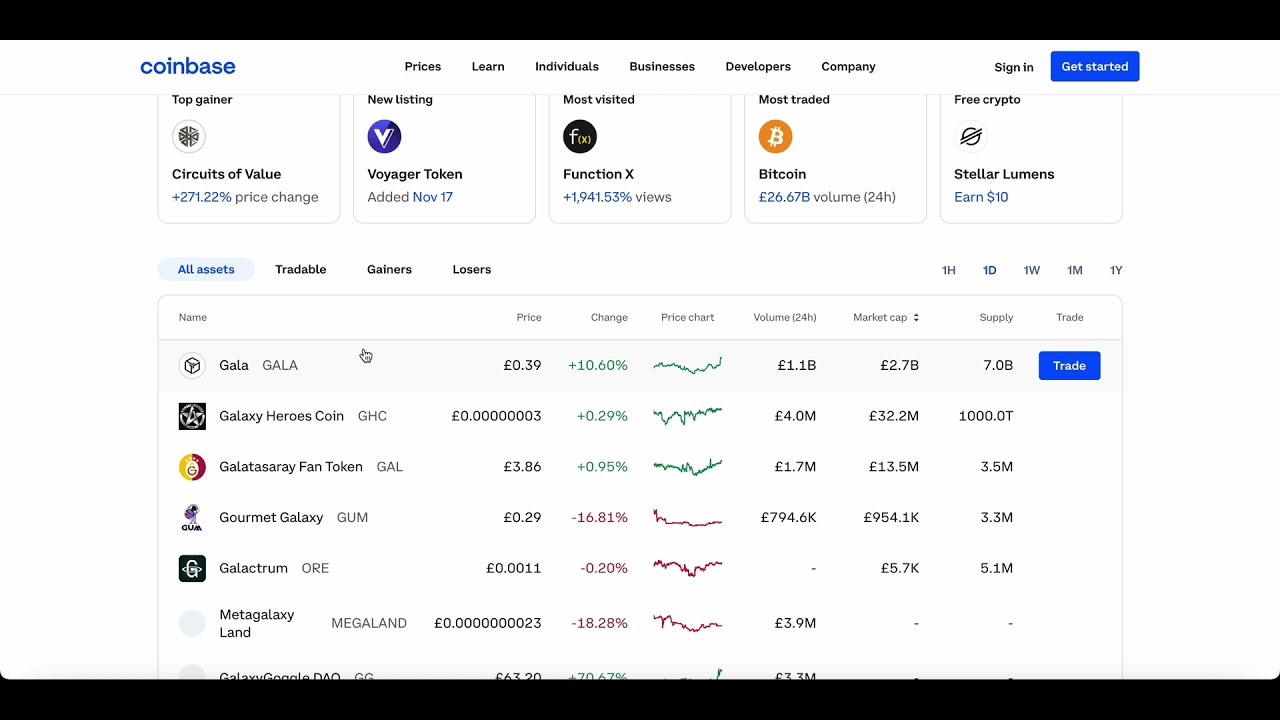The image is a screenshot of someone's computer or laptop screen, captured in a rectangular shape with a landscape orientation. The screenshot has narrow black borders at the top and bottom, but no side borders, and is set against a white background.

Underneath the top black border, a thin gray line stretches across the screen, creating a small white space containing some text. On the left side in blue font is the word "Coinbase." Centrally located is smaller, black font displaying menu items such as "Prices," "Learn," "Individual," "Businesses," "Developers," and "Company." To the right, there is a "Sign In" button and a blue rectangular box with white font that reads "Get Started."

Beneath this menu section, there are five rectangular-shaped boxes, each highlighting different features. These boxes include titles such as "Top Gainer" with "Circuits of Value," "New Listing" with "Voyager Token," "Most Visited" with "Function X," "Most Traded" with "Bitcoin," and "Free Crypto" with "Stellar and Lumens."

Below these feature boxes, a graph is displayed. This graph shows various items listed alphabetically, most starting with the letter "G." The columns include headings such as "Price Change" and "Price Chart," with data shown in green and black fonts to highlight gains and losses. Small images or icons are positioned to the left of each listed item, adding a visual element to the data presentation.